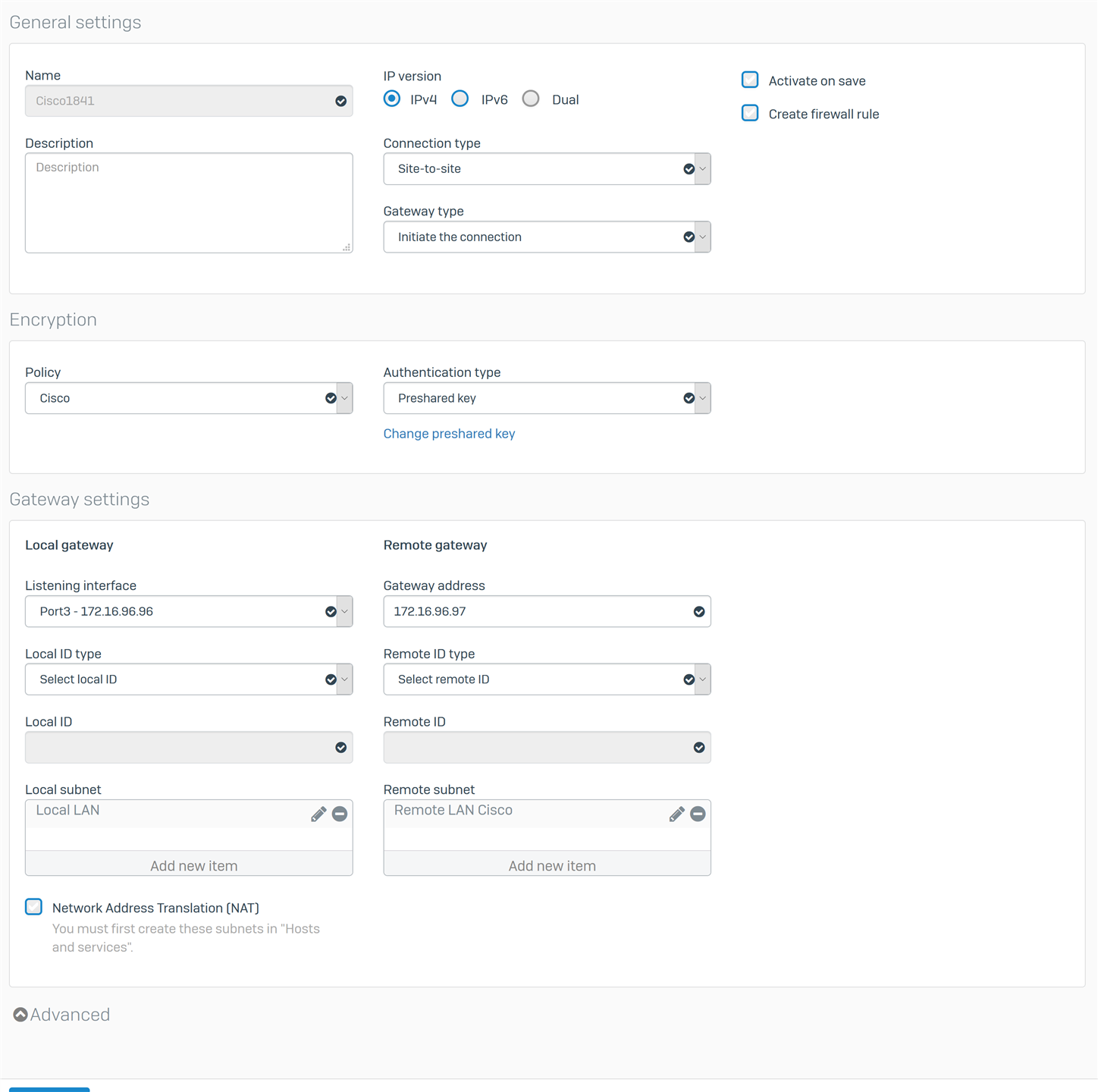This image displays a detailed configuration interface, primarily designed for network and security settings. At the top, there's a general settings section which includes a field for entering a name and a description box. To the right of these fields, there are options for selecting the IP version, with three available choices.

Below these settings is a section for specifying the connection type, and it's followed by options to select the gateway type. On the right side of this section, there is a checkbox labeled "Activate on save," and below that, another checkbox titled "Create firewall rule."

Moving to the next major section, the top left corner displays "Encryption." A gray dividing line runs horizontally underneath. This section includes a field labeled "Policy," which has a default value of "Cisco." To the right of the policy field, there is an "Authentication Type," set to "Pre-Shared Key," and an option to "Change Pre-Shared Key."

Following this, there is a "Gateway Settings" section. Under "Gateway Settings," there are multiple specifications: "Listening Interface," "Local ID Type," "Local ID," and "Local ID Subnet." Adjacent to these, on the right, are fields for "Gateway Address," "Remote ID Type," "Remote ID," and "Remote Subnet."

At the bottom, on the left, there's an option labeled "Network Address Translator" marked by a blue selection square.

This comprehensive interface is meticulously organized to allow for extensive customization and precise configuration of network parameters.